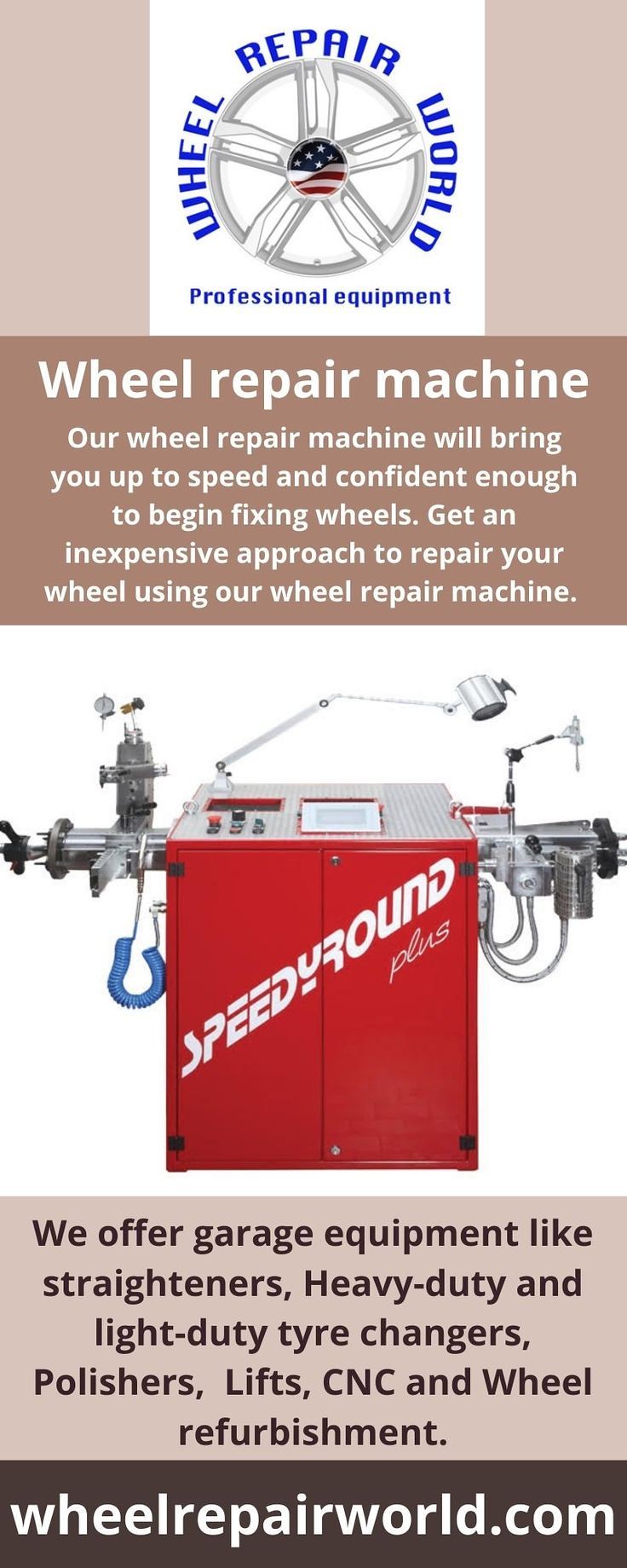The advertisement is titled "Wheel Repair World" and features a detailed central logo with a silver five-spoked wheel and an American flag in the middle. Below this, blue text reads "Professional Equipment," followed by white text that says "Wheel Repair Machine" against a brownish background. The ad promotes that their Wheel Repair Machine will make you confident and efficient in repairing wheels, offering an affordable solution. The core of the ad is a detailed image of the Wheel Repair Machine, branded as "Speedy Round Plus," characterized by a large red base with cabinet-like structures and a plethora of components such as wires, hoses, buttons, and tools. The bottom section presents black text on a tan background, listing various garage equipment like straighteners, tire changers, polishers, lifts, CNC, and wheel refurbishment. Finally, white text on a black background provides the website "WheelRepairWorld.com."